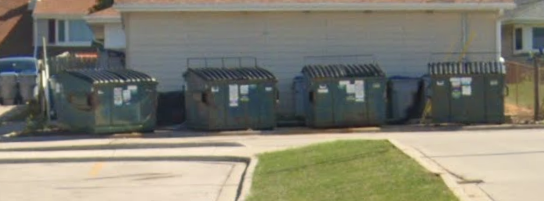The image depicts a row of four slightly beat-up blue dumpsters, each with hinged, split plastic lids, which are currently closed. These dumpsters, adorned with various stickers and white papers, are positioned under an awning attached to a block brick building with light-colored siding. Surrounding the dumpsters are several smaller garbage pails, also covered with flap-like lids. In front of the setup, there’s a strip of mown grass, bordered by a parking lot with concrete sidewalks and visible curbs. The scene includes additional background elements: a chain-link fence behind the brick building, residential homes on either side, and a passenger vehicle visible on the left. The area suggests shared use of dumpsters, potentially by multiple households.